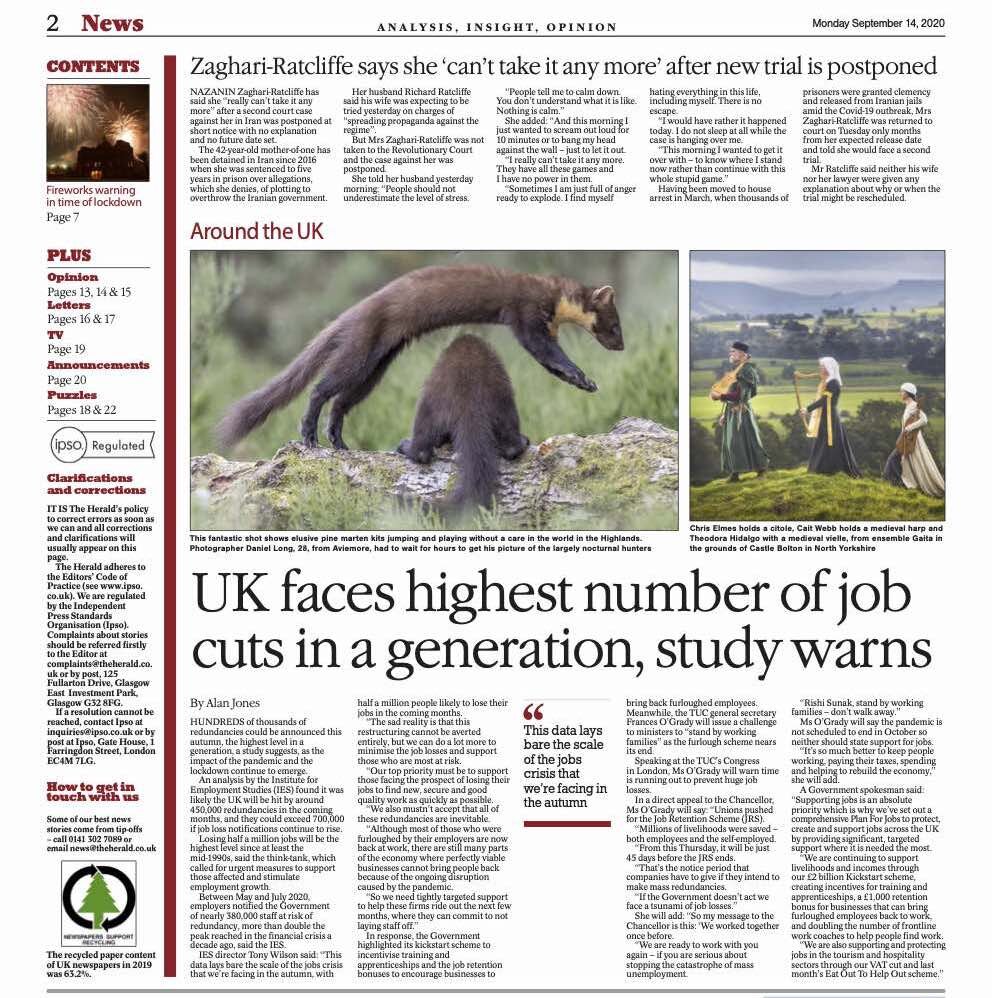The newspaper article displayed has a slightly gray background and various elements meticulously arranged throughout the page. In the top left corner, a black number "2" is prominently positioned, followed by a thin, black horizontal line that spans the entire width of the page. To the right of the number, "NEWS" is written in red text. Centrally aligned are the words "ANALYSIS, INSIGHT, OPINION" in bold, uppercase black text. On the far right, the date "MONDAY, SEPTEMBER 14, 2020" is presented in small sans-serif black text.

On the left side of the page, there is a sidebar containing rows of text and an image of fireworks at the top. Above the fireworks image, the word "CONTENTS" is printed in red text. A thick, dark red vertical line runs the full length of the page, separating the sidebar from the main article.

Beneath the header line and adjacent to the top of the dark red line, the headline "ZAGARI RATCLIFFE SAYS SHE CAN'T TAKE IT ANYMORE AFTER NEW TRIAL IS POSTPONED" is displayed prominently. The main body of the article follows, formatted in small text with paragraphs typically spanning 2-3 lines each. Further down, aligned to the left, the section titled "AROUND THE UK" is highlighted in red text.

Below this section, two photographs are positioned side by side, each framed with a thin black outline. The left photograph captures two martens: one facing away and sitting on a log with its tail draped over it, and another mid-leap, arching over the first. The right photograph depicts three individuals clad in medieval attire, carrying medieval instruments, and walking across a vibrant green hill with a valley and mountains in the distant background. Each photograph is accompanied by a small caption beneath it.

At the bottom of the page, a bold, large headline states, "UK FACES HIGHEST NUMBER OF JOB CUTS IN A GENERATION, STUDY WARNS."